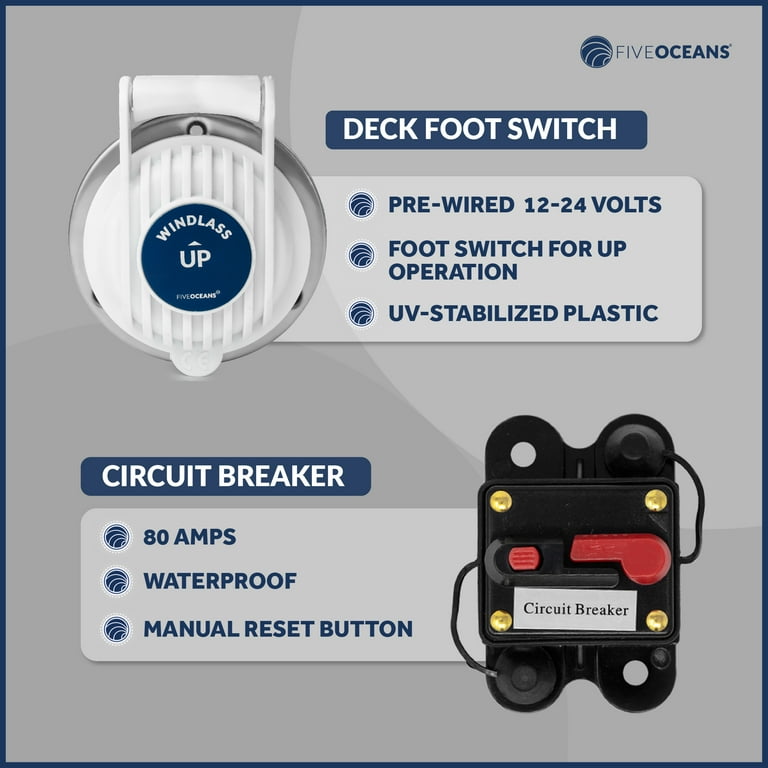The digital advertisement poster features detailed information about two marine electrical products against a grey background with a blue border. Near the top left side of the poster, there is an image of a round, white electric switch with a silver metallic part in the middle. Attached to it is a blue sticker with the text "Windlass Up." To the right of this switch, descriptive text reads: "Deck Foot Switch, Pre-wired 12 to 24 volts, Foot switch for up operation, UV-stabilized plastic."

In the bottom right side of the poster, another image displays a black circuit breaker with red components in the middle and golden screws at the corners. A sticker on this circuit breaker clearly labels it as "Circuit Breaker." The adjacent text further explains: "Circuit breaker, 80 amps, waterproof, manual reset button."

At the top right corner, the brand logo "5 Oceans" is prominently featured. All text on the poster is written in either white or blue, tying into the color scheme. This visually appealing advertisement effectively highlights the Deck Foot Switch and Circuit Breaker, making it easy for potential buyers to understand their features and benefits.